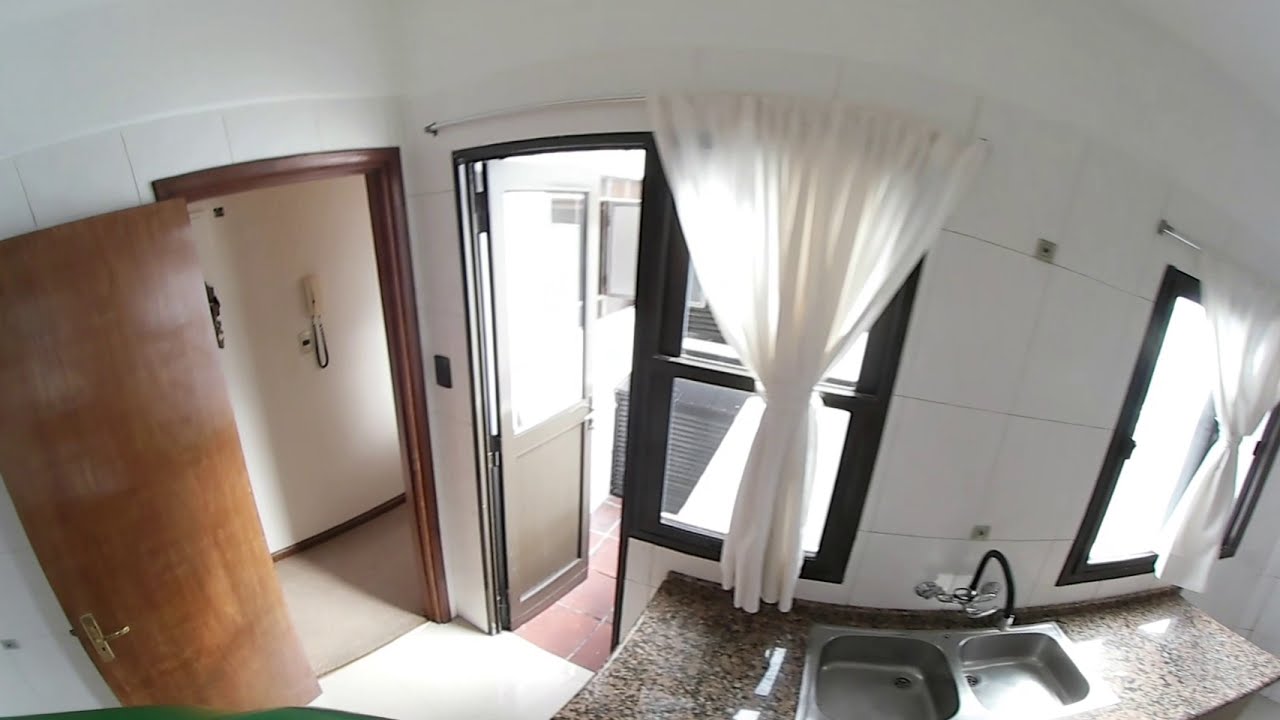This image depicts the interior of a kitchen area, possibly part of a house or apartment, captured from a high vantage point suggesting a viewpoint like that of a security camera. The space features a countertop made of black and brown speckled granite with a built-in double stainless steel sink and a distinctive black loop-design faucet extending from the wall. 

Above the sink, two black-framed windows allow sunlight to filter through, illuminating the room. These windows are adorned with white curtains tied in the middle, contrasting with the large white tiled walls. The kitchen has a significant source of natural light, indicated by the bright daylight streaming through the windows.

To the left side of the image, there's an open wooden door that appears to lead to a hallway, where a corded phone is mounted on the wall. Adjacent to this door is another door, potentially made of aluminum, that is open to a small balcony area paved with red square concrete tiles. Inside the kitchen, the floor features a mix of white tiles and a gray carpeted area. The ceiling is white, complementing the overall light and airy atmosphere of the space.